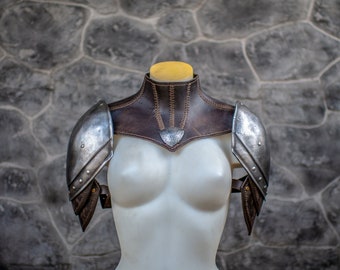This photograph features a headless mannequin styled to resemble the torso of a woman, positioned against a gray stone wall. The mannequin has a detailed white body with prominent breasts, a thin waist, and defined ribs. The display cuts off at the neck, with the upper chest and neck area extending to a light brown leather piece that covers from the upper chest to the neck. At the top of the neck, there's a yellow dot simulating where the head would be. The mannequin is adorned with metal shoulder armor, featuring silver or metal plates draped across the shoulders and extending slightly down the arms. The overall appearance gives the impression of a breasted woman warrior in partial armor, standing in a dignified pose despite the absence of a head.